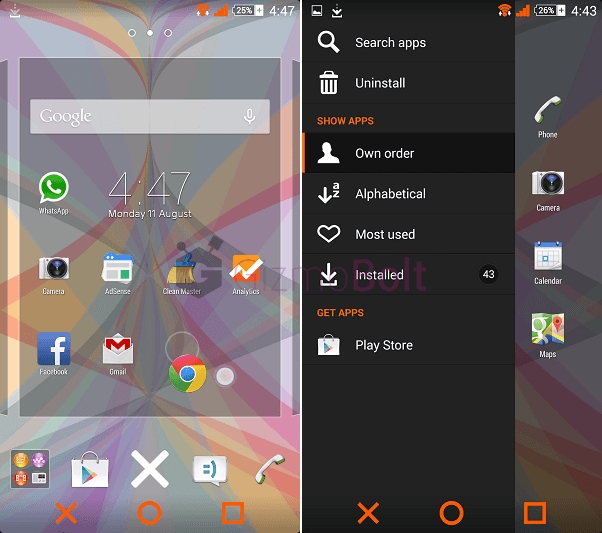The image displays two cellphone screenshots side-by-side. The screenshot on the left shows an app management interface, where users can organize their home screens. This interface allows for the customization of app placement across different screens. The interface features a grid-like arrangement where users can drag and move apps from one screen to another. Notably, there are three dots at the top, which indicate the presence of three different screens available for customization.

The screenshot on the right depicts an opened menu that has slid out from the left side of the screen. The menu starts with a "Search Apps" feature at the top, followed by a list of options: "Uninstall," a section called "Show apps" that includes options for "Own order," "Alphabetical," "Most used," and "Uninstalled." At the bottom, there is a section titled "Get Apps," featuring the Play Store icon, suggesting a link to Google's app marketplace.